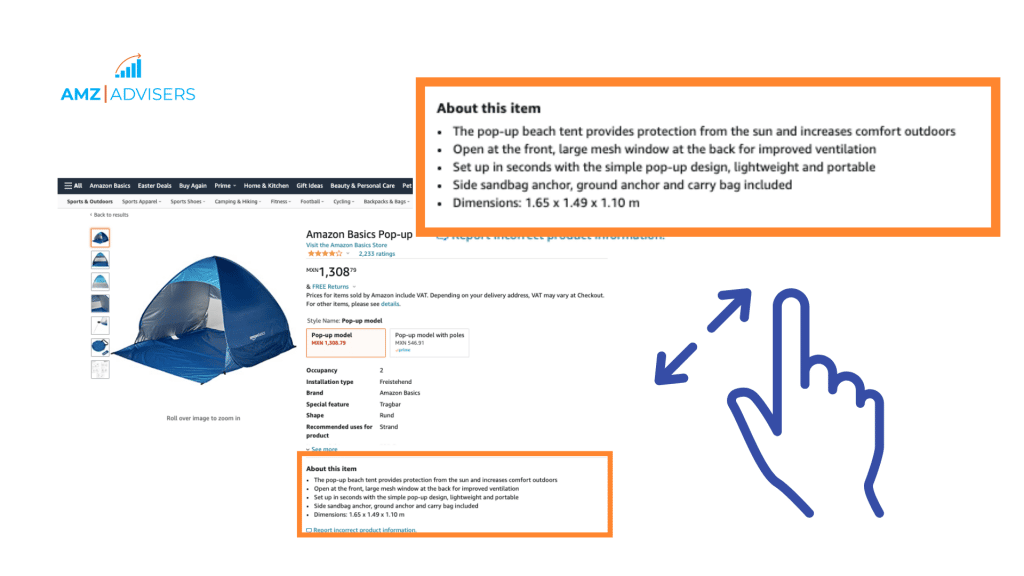In the upper left corner of the image, there’s a light blue logo with the text "AMZ Advisors". Below the logo, a computer screen is prominently displayed, showcasing an Amazon webpage. In the upper right corner of the screen, there’s an orange-outlined pop-up box, which has been zoomed in to highlight its content. To the side of this pop-up, there’s an icon depicting a gesture of a pointer finger and thumb moving apart, indicating a zoom-in action.

The pop-up box contains a section titled "About this item", followed by several bullet points detailing a product:

- The pop-up beach tent provides protection from the sun and increases comfort outdoors.
- Open at the front, with a large mesh window at the back for improved ventilation.
- Sets up in seconds with a simple pop-up design; lightweight and portable.
- Includes side sandbag anchors, ground anchors, and a carry bag.
- Dimensions: 1.65m x 1.49m x 1.10m.